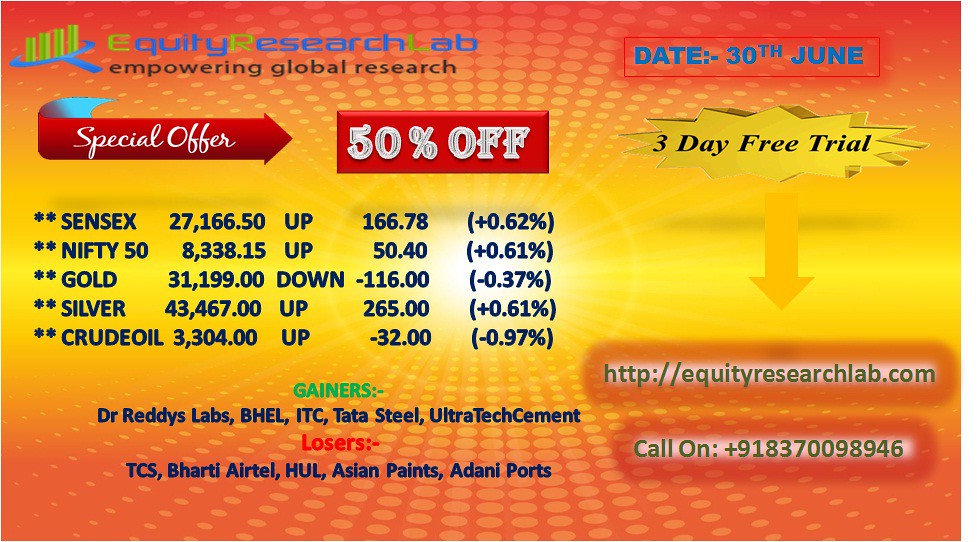The image appears to be a colorful advertisement, primarily featuring shades of orange and yellow with black and blue lettering. In the upper left-hand corner, the text "Equity Research Lab" stands out, with the first letters in light green and the rest in blue, alongside their tagline, "Empowering Global Research." Moving to the upper right, there is a date, "30th June," followed by a "Three-Day Free Trial" in black against the yellow background. Below this, a red banner with white text announces a "Special Offer," pointing to a red rectangle that reads "50% off" in white script.

The central portion of the advertisement lists various market data, including prices for Sensex, Nifty 50, gold, silver, and crude oil, each accompanied by its current price and a percentage change indication. For instance, Sensex is noted to be up 166%, Nifty 50 up 50%, gold down, silver up, and crude oil with respective values such as gold at $31,199 and silver at $43,467. Below this data, gainers are listed in green, naming companies like Dr. Reddy's Labs, BHEL, ITC, Tata Steel, and Ultra Tech Cement. Conversely, in red, the losers include TCS, Bartle, Airtel, HUL, Asian Paints, and Adani Ports.

Lastly, in the lower right-hand corner, the website "EquityResearchLab.com" and a phone number are provided, completing the detailed and vibrant layout of this advertisement.